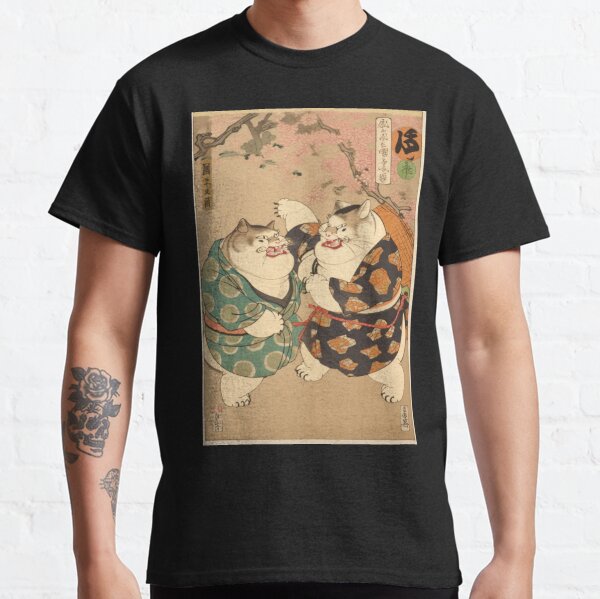In front of a white brick wall stands a young man wearing a black, short-sleeved t-shirt adorned with a vibrant and detailed graphic. The centerpiece of the shirt is a rectangular image featuring two white-furred, somewhat obese cats, each clad in traditional Japanese kimonos. The cat on the left is dressed in a green kimono, while the one on the right sports a black and orange kimono. They appear to be engaged in a dynamic, combative pose, facing each other. Above the cats, in the top right corner of the graphic, are Asian characters rendered in a calligraphic style, adding to the Japanese-themed aesthetic. The man has peach-colored skin and a distinctive tattoo of a rose in a glass on his right forearm. His left arm, devoid of tattoos, is visible alongside his neck, which is centered at the top of the image. The overall photograph seems to focus on showcasing the screen-printed design of the t-shirt.